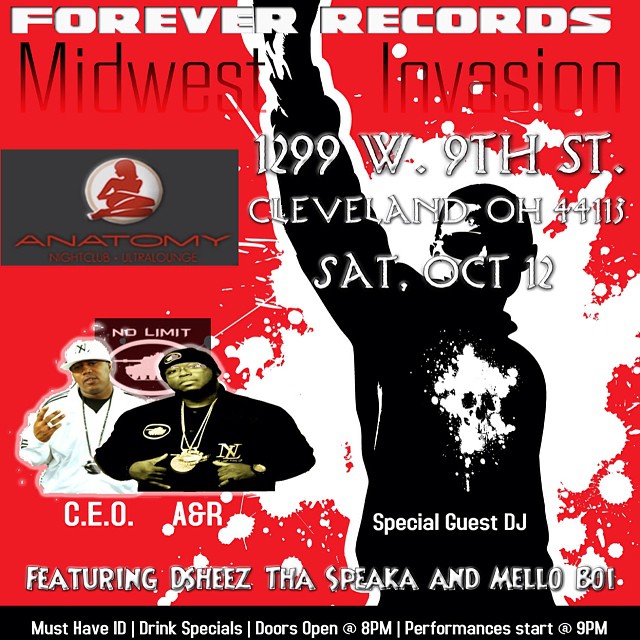This detailed promotional poster for the event "Midwest Invasion," presented by Forever Records, advertises a night of musical performances at the Anatomy Nightclub Ultra Lounge, located at 1299 West 9th Street, Cleveland, Ohio 44113. The event takes place on Saturday, October 12th, with doors opening at 8 p.m. and performances starting at 9 p.m. The poster prominently features photographs of two individuals labeled 'CEO' and 'A&R', alongside a drawing of a special guest DJ in a skull t-shirt. Additional featured musicians include Dee Shees, The Speaka, and Mellow Boy. The background of the advertisement is red, with white splatter behind a silhouette of a person raising their hand on the right side. Attendees must present ID, and there will be drink specials available. The logo of the Anatomy Nightclub, showing a woman sitting down, is displayed on the left-hand side of the image.